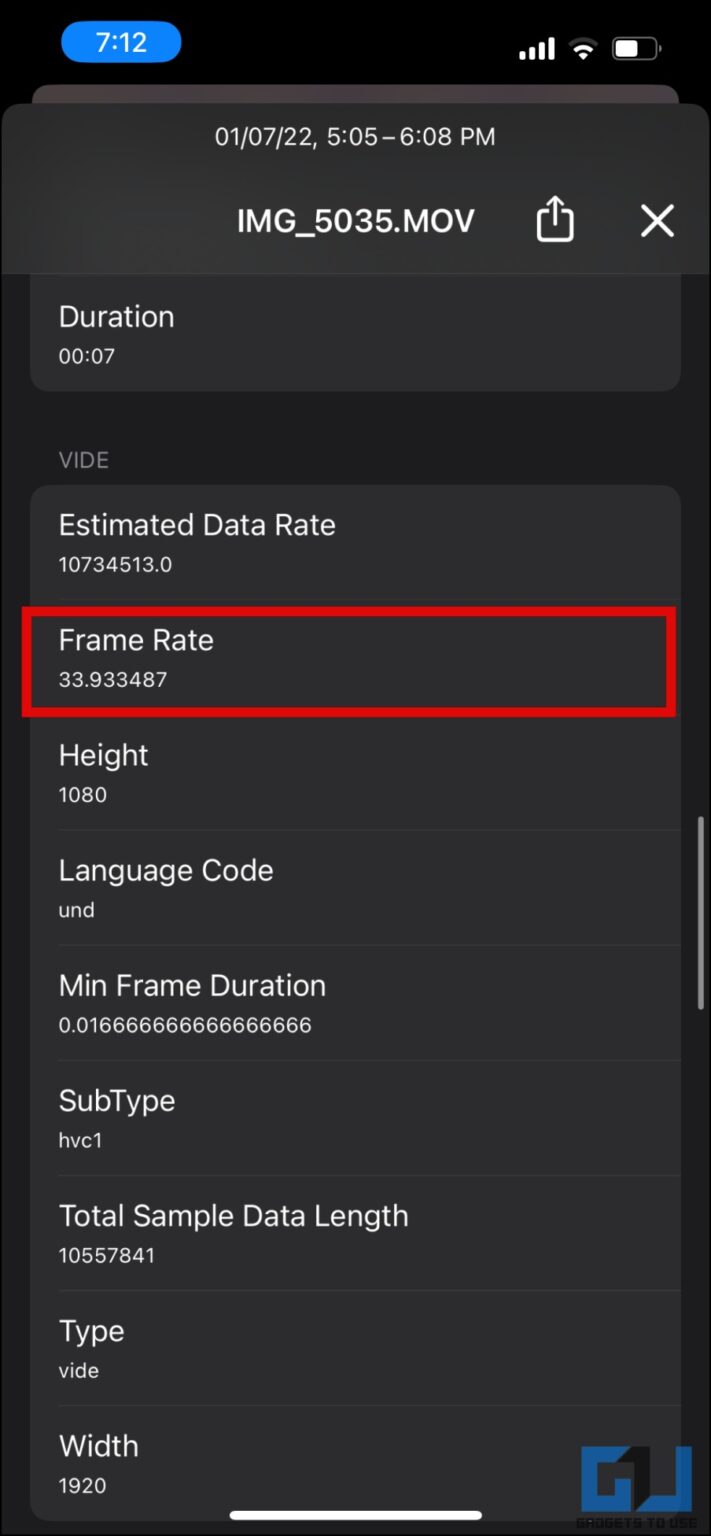The image features a black background with a prominent screen display. In the bottom right-hand corner, there are two block-style, three-dimensional letters: a bright blue "G" and an adjacent backward capital "L," both outlined in black. The screen displays the file name "IMG_5035.MOV" alongside various metadata. This includes details such as the duration, estimated data rate, frame rate (33933487), height, language code, minimum frame duration, subtype, total sample date length, type, and width. All the information is printed in white text, enclosed within a red rectangular box that spans across the screen, including the empty spaces.